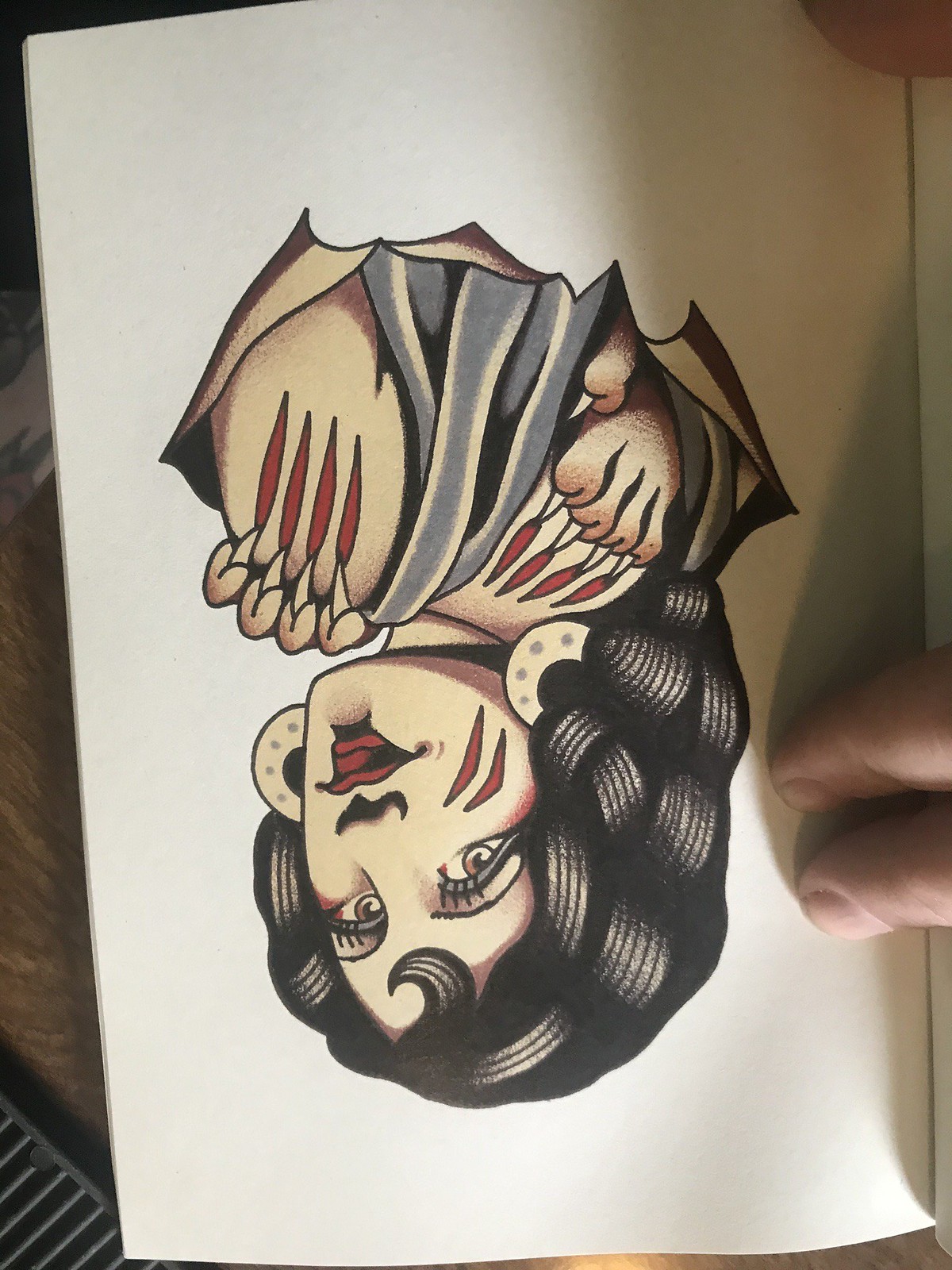In the photograph, a meticulously detailed drawing is placed upside down on a wooden floor. The floor displays a visible metal grate where air flows through, adding to the realistic setting behind the artwork. Two fingers are seen gently touching the edge of the drawing, perhaps suggesting admiration or curiosity. The drawing itself portrays a female character, rendered in an anime-inspired style. She has long, flowing dark hair and captivating pale brown eyes, accentuated by her prominent eyelashes. Her look is further enhanced with red lipstick that gives her lips a slightly pouty appearance. Intriguingly, her hands are depicted as claws, leaving visible scratch marks on her shoulder, one direction. She adorns gold hoop earrings and has a gray drape elegantly resting on her shoulders. This illustration is a unique creation by an artist.